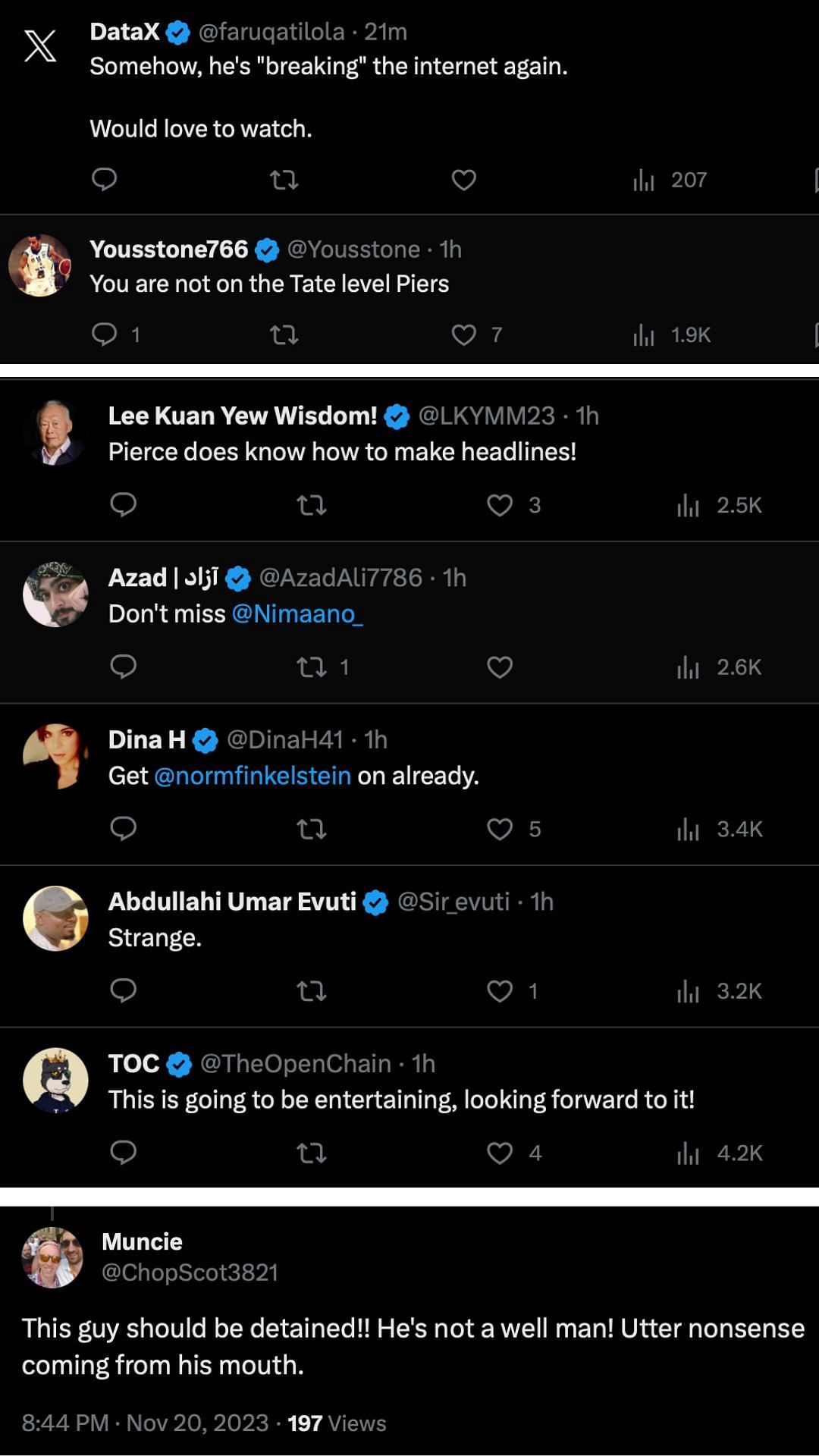The image depicts a collection of tweets on the X platform, captured in "midnight mode" for a dark-themed background with white text. 

- The first tweet is from DataX at Fort Quatolia, posted 20 minutes ago, stating, “somehow he's breaking internet again. Would love to watch.” 
- Stone776 replied an hour ago saying, “You are not Tate level of peers,” receiving one comment and seven upvotes.
- LeeConYouWisdom also commented an hour ago, “Pierce does not know how to make headlines,” garnering three likes. 
- Azjad Ali, tweeting at @AzjadAli7786 an hour ago, mentioned, “Don’t miss it, Naimo,” with one quote reply but no likes.
- Deena H, @DeenaH41, urged, “Get Nam Finkelstein on already,” and her tweet received five likes.
- Abdullah Umar Ivedi, identified by @SirIvedi, simply commented, “Strange,” which had one like.
- Tak The Open Chain responded with anticipation, stating, “This is going to be entertaining. Looking forward to it,” earning four likes.
- Below these interactions is a tweet from Muncy, posted at 8:44 PM on November 20th, 2023, with 197 views: “This guy should be detained. He's not well, man. Utter nonsense coming from his mouth.”

Each tweet includes a distinctive avatar, ranging from portraits of people to whimsical images like a dog with a crown, a testament to the personalized nature of profile pictures on social media.